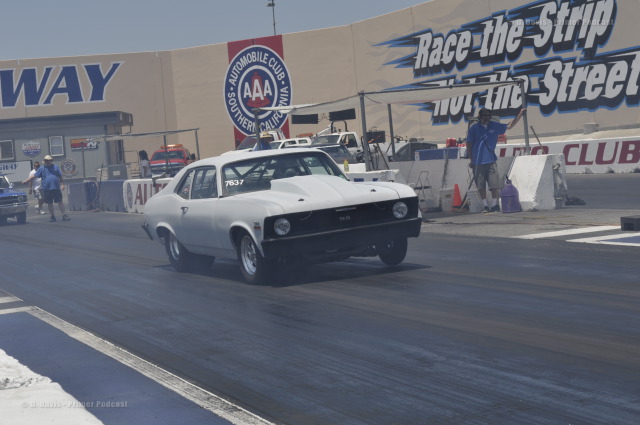The image features a vintage white muscle car, likely from the 70s or 80s, aggressively accelerating off the starting line on a drag strip. The car's powerful launch is evident as its front wheels, especially the front left, are lifted off the ground, suggestive of its intense speed and vigorous grip on the roadway. The dark black asphalt contrasts with the vibrant scene. Behind the action, a building bears a prominent circular logo of the AAA Automobile Club of Southern California, accompanied by the striking white text "Race the Strip, Not the Street," embellished with blue flame graphics to add a dramatic flair. The drag strip is bustling with activity, including race officials and attendants clad in blue shirts, some wearing shorts and others in pants, and hints of smoke in the air, adding to the high-octane atmosphere. In the backdrop, a little blue car appears poised, likely as the next racer to take to the strip. The scene captures the raw energy and excitement of a drag racing event.